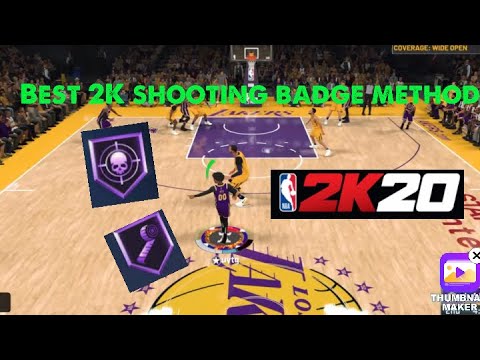The image is a screenshot from the NBA 2K20 basketball video game, presented in landscape orientation, likely captured on a tablet. The image features letterbox framing, with dark black bars across the top and bottom. On the right side, approximately halfway down, there is a black rectangle that contains the NBA logo with a dribbling player, accompanied by "2K20" in thick, italicized red and white letters.

In the bottom right corner, the name "Thumina Maker" appears, which may be the player's name. The court depicted is a light wood basketball court with a yellow boundary and an LA Lakers logo at its center. The phrase "Best 2K Shooting Badge Method" is prominently displayed in large green letters across the top of the image.

The scene shows a crowd watching a basketball game from a midcourt perspective, looking towards a basket. Players are highlighted with circles around them. A Lakers player is visible with the number 00 on their purple and gold jersey. There are also two blue square boxes on the screen, resembling cards or action icons. The top box has a shape similar to a baseball base with a crosshair and skull symbol inside, while the bottom box contains an unidentified icon that could resemble a measuring tape or basketball.